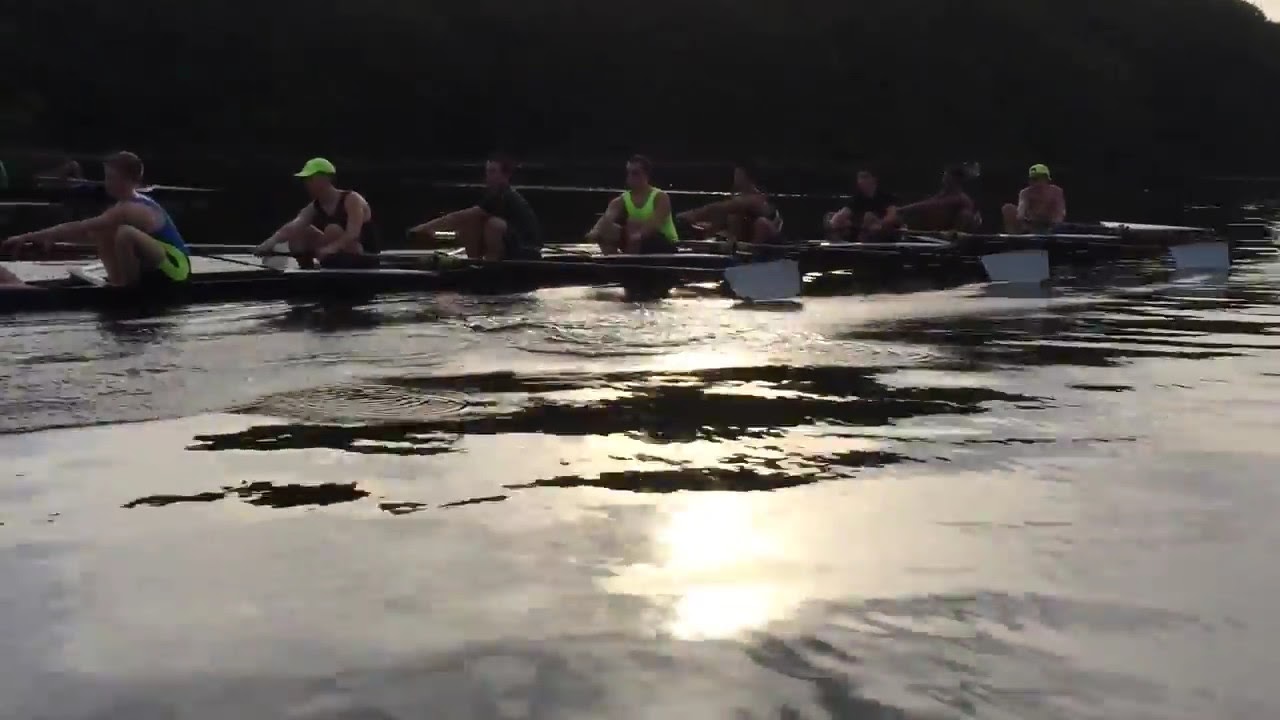In this image, we observe a group of people canoeing together on a body of water, likely a lake or river. The scene captures a total of eight visible individuals in two different canoes, with a possible ninth person in the distance. Many of the participants appear to be wearing light-colored clothing, which enhances their visibility. Notably, one person sports a lime green hat, while another is dressed in a matching neon green tank top. The majority of the group seems to be male, enjoying an outdoor adventure.

The water beneath them ripples gently, reflecting the sunlight that pierces through to the middle area, indicating that it's early in the day with the sky not yet fully bright blue. In the background, darker areas suggest the presence of trees, adding contrast to the vibrant activity on the water. Among the rowers, there's a distinct sequence of attire: starting from the left, the first individual wears a blue shirt with green pants, followed by several others in black shirts and black pants. Interestingly, the last person is shirtless with black pants. Though most appear to be male, there is some uncertainty about the second-to-last rower, who might be female or simply have darker skin, as it’s difficult to discern from the shadows.